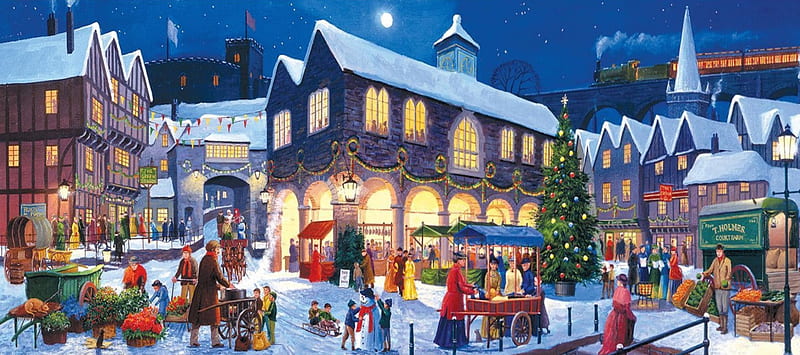This animated scene captures a bustling holiday evening in a town square brimming with activity. The focal point is a large, two-story building adorned with wreaths and garlands, featuring grand archways on the first floor and tall arched windows on the second. A white steeple rises from its roof, facing slightly to the right. A festive Christmas tree, topped with a radiant white star, stands proudly in front of this central building. The town square is alive with people—some gathered by small market stands selling produce and flowers, others near a little stand in the center. On the bottom left, a flower stall is surrounded by onlookers, while on the bottom right, a fruit and vegetable vendor serves customers. Snow blankets the rooftops of Bavarian-style houses flanking the scene, and children can be seen playing and building snowmen. The night sky above, adorned with stars and a bright moon positioned above the central building, adds a magical touch. In the distance on the right, a train travels from left to right over a large brick bridge, completing this charming winter tableau.